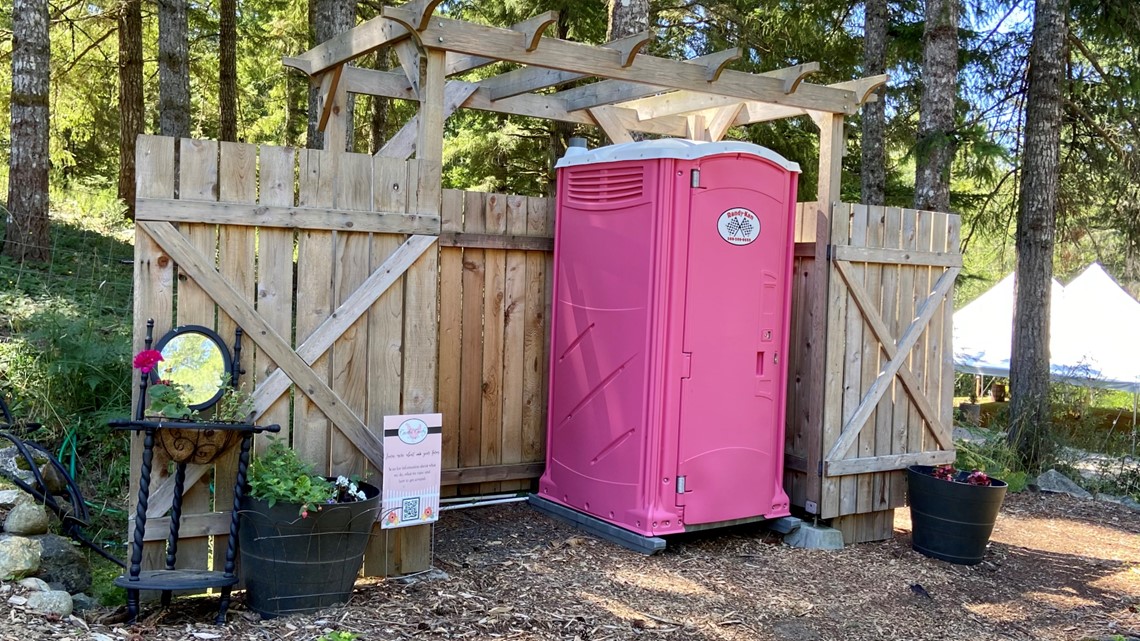In this sunny, nature-filled setting, a pink port-a-potty with a white roof stands prominently against a wooden structure that forms a partially open roof and walls. The wooden structure features a circular mirror and a three-legged black stool, adorned with a red flower and two green plants. Near this setup, a potted plant rests on the ground, along with a small pink sign or card that is difficult to read from this distance. The front of the port-a-potty displays a logo with two crossed racing flags. Surrounding the scene, we see trees and a white pop-up event tent, indicating a forest or campground location. The brown ground and clear sky further emphasize the outdoor, sunny ambiance of the image.